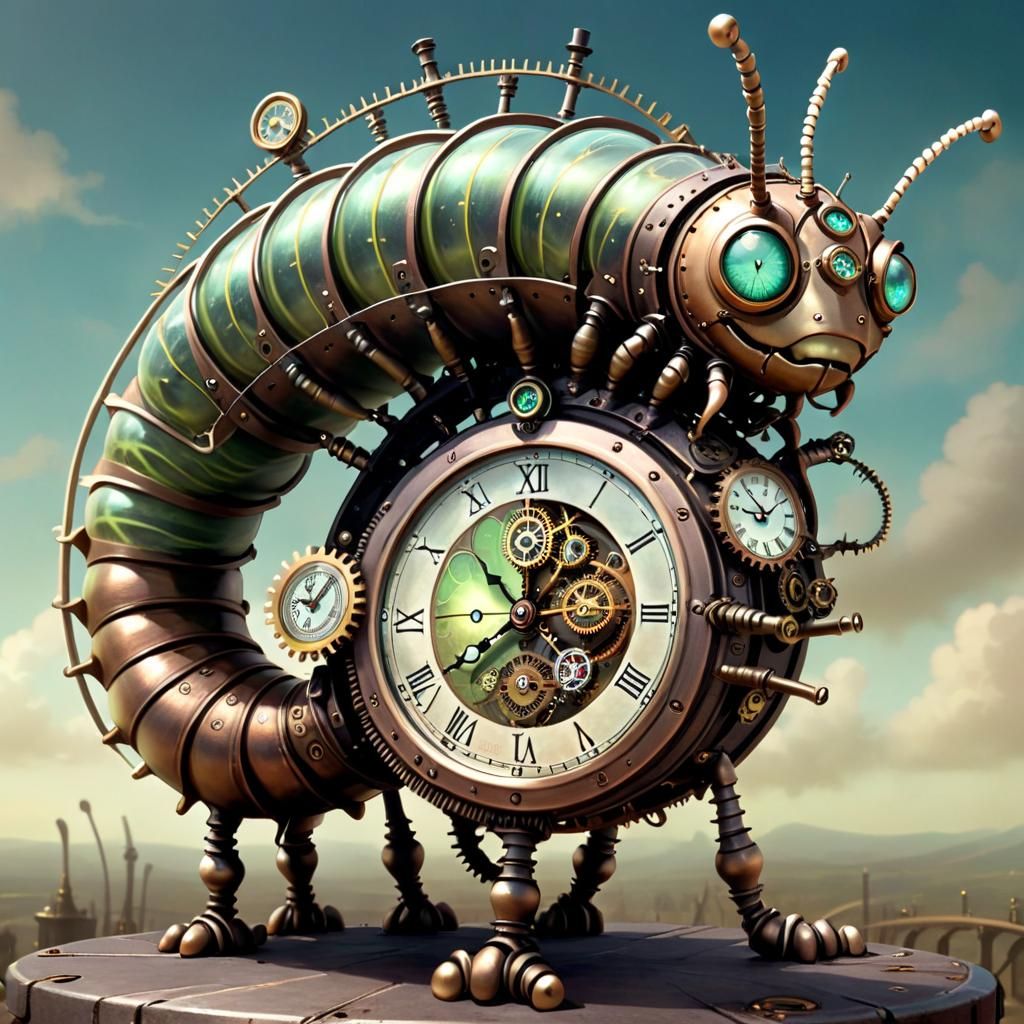The image depicts a highly detailed, computer-generated graphic of a steampunk-inspired mechanical caterpillar that merges elements of a clock and a robotic creature. Its body, made of copper and green metallic material, features a central clock with Roman numerals and visible gears. The caterpillar has six metallic legs supporting it. Its body emerges from the left side of the clock, curves around and over it, ending near its face which has multiple bluish-green, shiny eyes. The face also has three antennas and a brass appearance. Additional smaller clock faces adorn its sides. A spine-like structure with a gauge runs along its back. The mechanical caterpillar stands on what appears to be a metal stand or manhole cover, against a backdrop of mountains and a cloudy sky. The image displays some AI-like qualities, suggesting it was generated digitally.